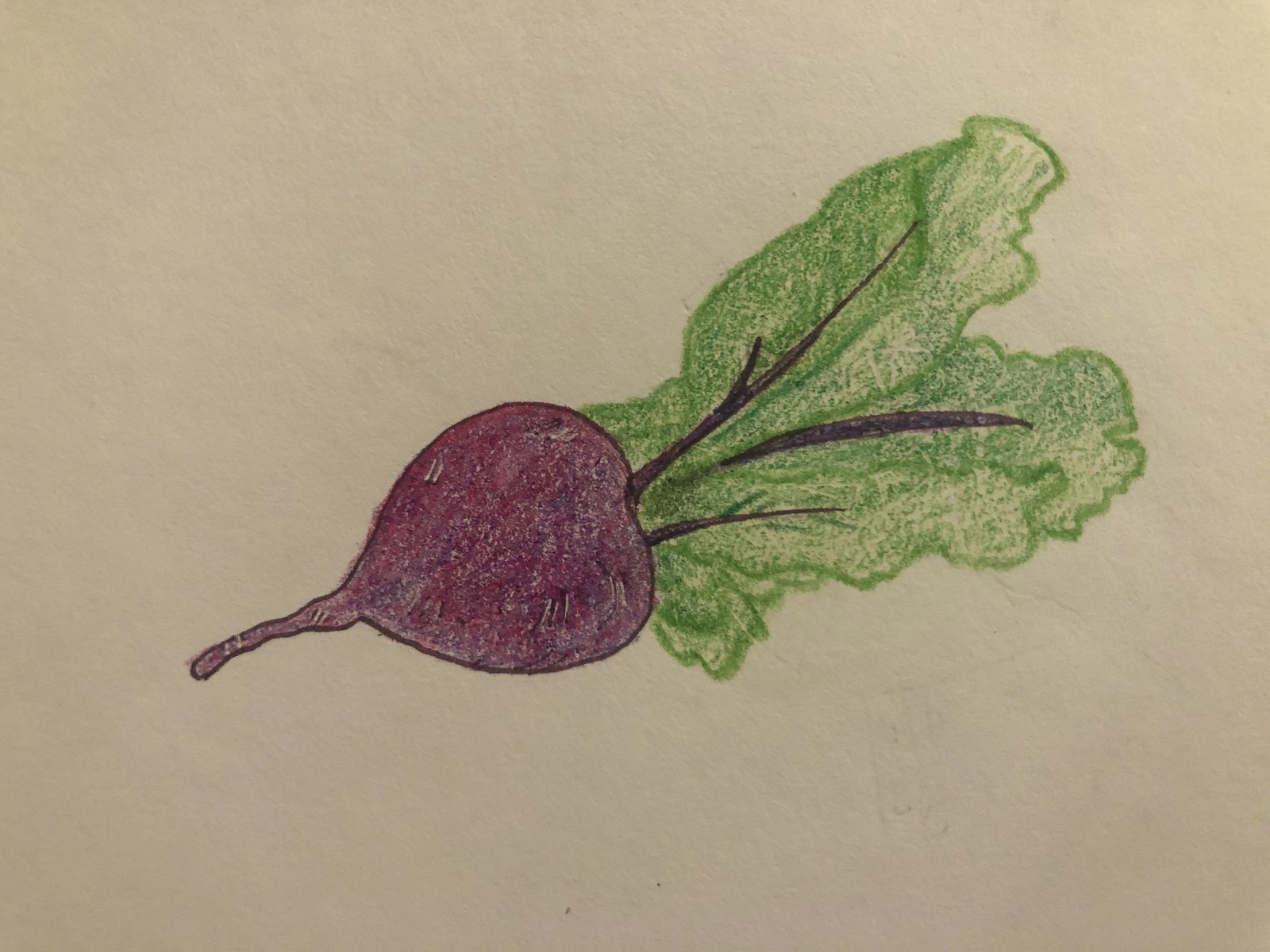This image features a highly detailed drawing on a cream-colored piece of paper. At the center of the composition lies a vegetable that closely resembles a beet, characterized by its deep purple, burgundy-maroon hue. The vegetable is nearly circular with a small, tapering tail extending from one end. The green leaves, attached to the right side of the bulb, are meticulously illustrated to show their veins and stems, suggesting a realistic texture despite being colored in a crayon-like manner. The paper background exhibits a subtle gradient, with a slightly darker tinge on the left side compared to the lighter right side. Overall, this detailed drawing skillfully captures the intricate features of the beet and its foliage, with the leaves pointing to the right and the bulb's tail extending to the left.